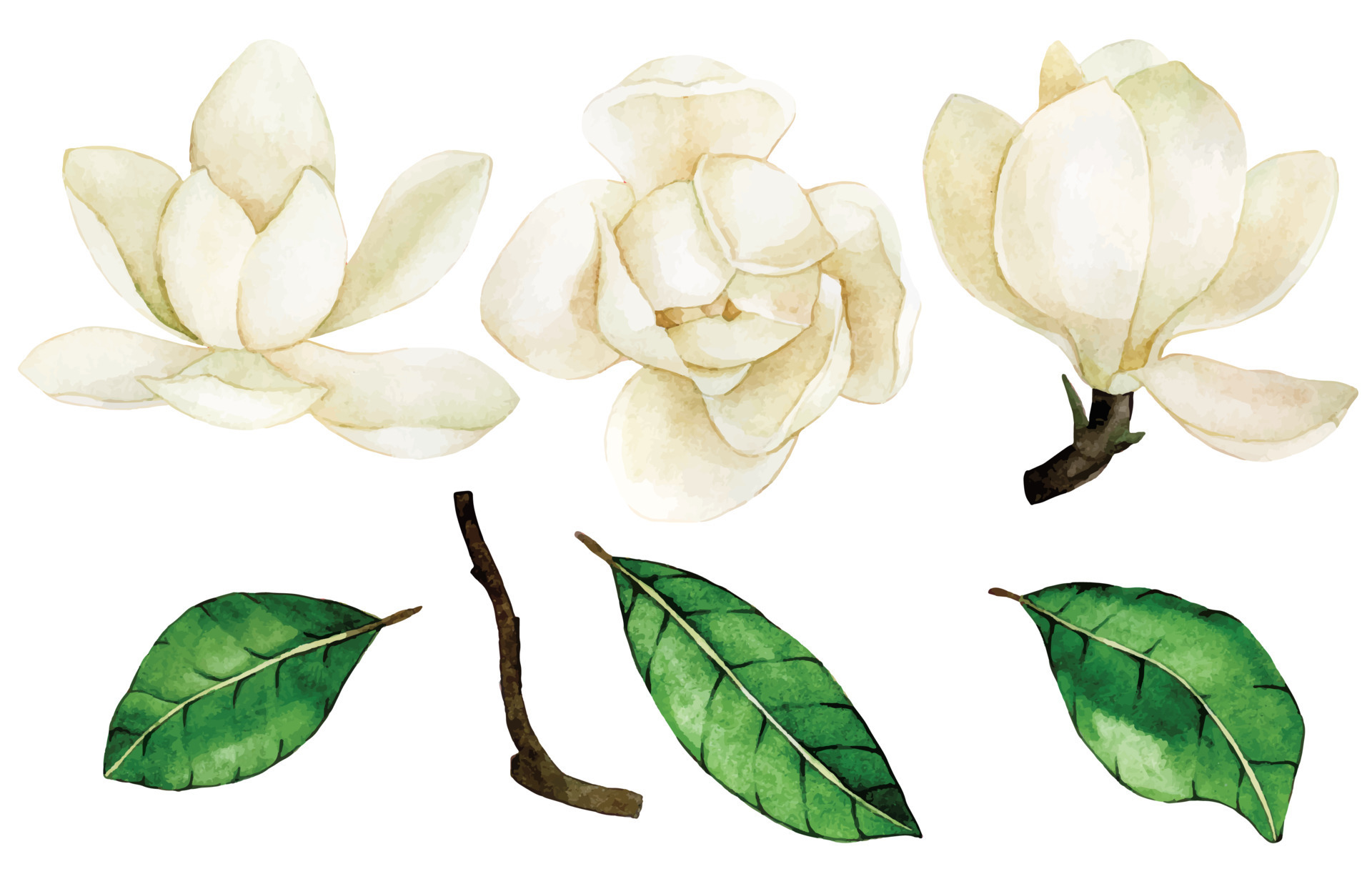This detailed botanical illustration captures the various perspectives of a white flower with intricate shading. 

- **Left Image**: A side view of the partially disassembled flower, showcasing a few petals detaching from the main structure.
- **Middle Image**: A top-down view of the flower, highlighting its semi-bloomed state with most petals still attached.
- **Right Image**: Another side view featuring one petal falling off and a glimpse of the stem.
- **Bottom Image**: An arrangement consisting of a solitary stem flanked by three detached leaves, which are prominently green with visible veins.

The entire drawing emphasizes the flower's delicate structure through meticulous shading and detail.